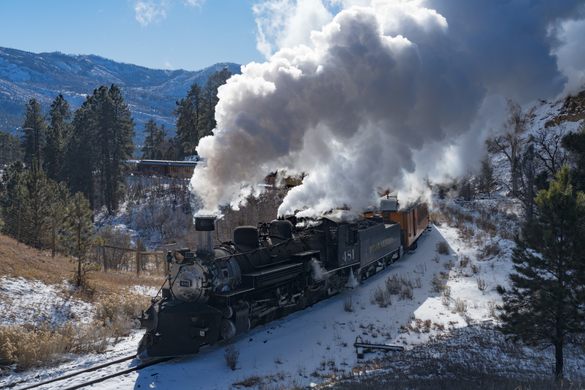This image captures a nostalgic scene of an old-fashioned steam engine train racing down the tracks in a high-elevation, snowy landscape. The train, predominantly black and gray, emits billowing clouds of white and gray smoke, creating a dramatic contrast against the crisp light blue sky. To the right of the train, the ground is covered with sparse snow patches interspersed with grass and shrubbery, while the left side has less snow, revealing more grass. The train is pulling a series of passenger cars, primarily brown with gray roofs, that stretch far into the background. Surrounding the scene are bluish-hued mountains and dark green evergreen trees. The train's track curves slightly, adding a dynamic sense of motion to the photograph. The presence of snow, the mountains, and the evergreen trees suggest this is a picturesque countryside setting in colder weather, with the sunlight more prominent on the left-hand side of the image.